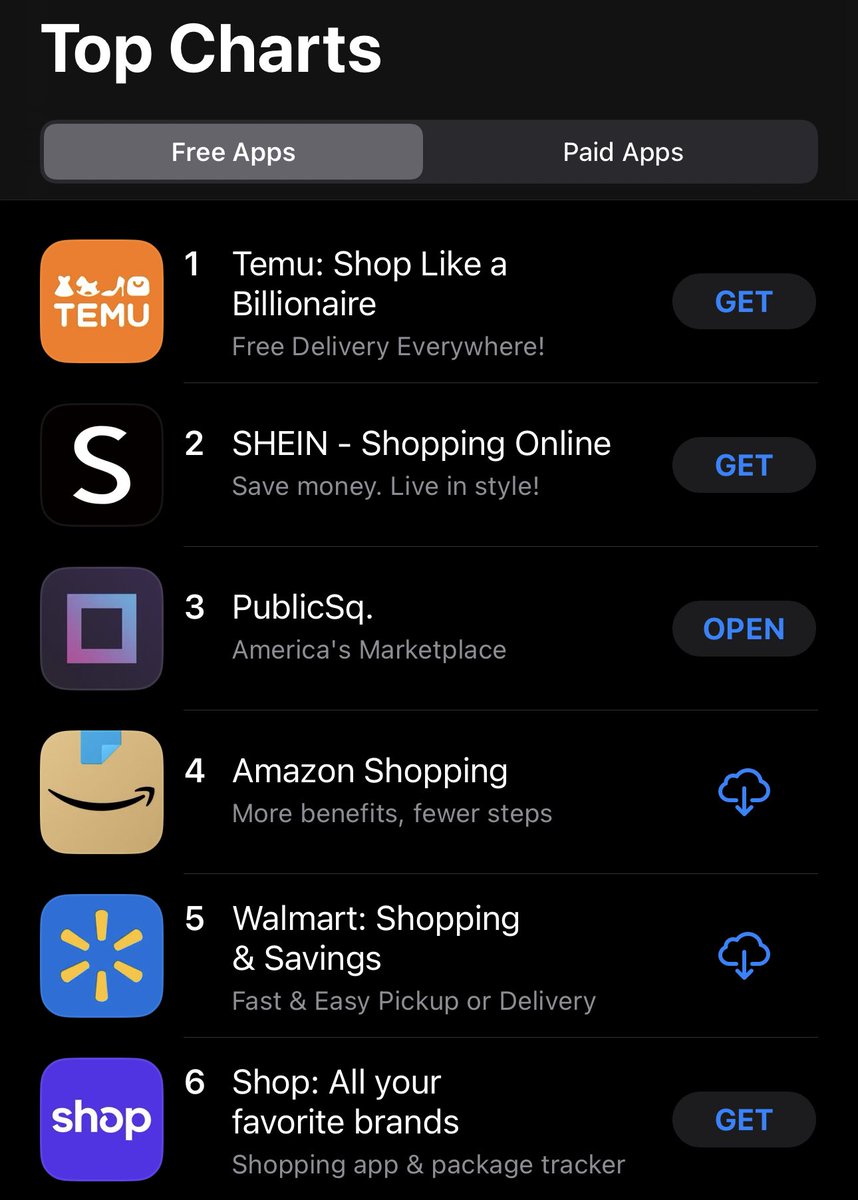A screenshot of the Apple App Store showcased in dark mode. The screen is displaying the "Top Charts" section, particularly the "Free" category within the shopping genre. The top six free apps are listed as follows: Temu, Shein, PublicSq (Public Square), Amazon Shopping, Walmart, and another unnamed app promoting shopping for favorite brands. Temu and Shein feature a "Get" button, indicating that they have not been previously downloaded. Amazon Shopping and Walmart display a cloud icon with an arrow, suggesting they were downloaded before and can be re-downloaded. PublicSq is already installed, evident by the "Open" button beside it.

The interface is minimalistic with a dark theme, utilizing white and gray font colors, while buttons are highlighted in blue. This layout highlights the popularity of these shopping applications, including notable Chinese platforms like Temu and Shein. The overall design is clean and straightforward, which helps emphasize the prominence and user engagement with these top-charting apps in the shopping category.